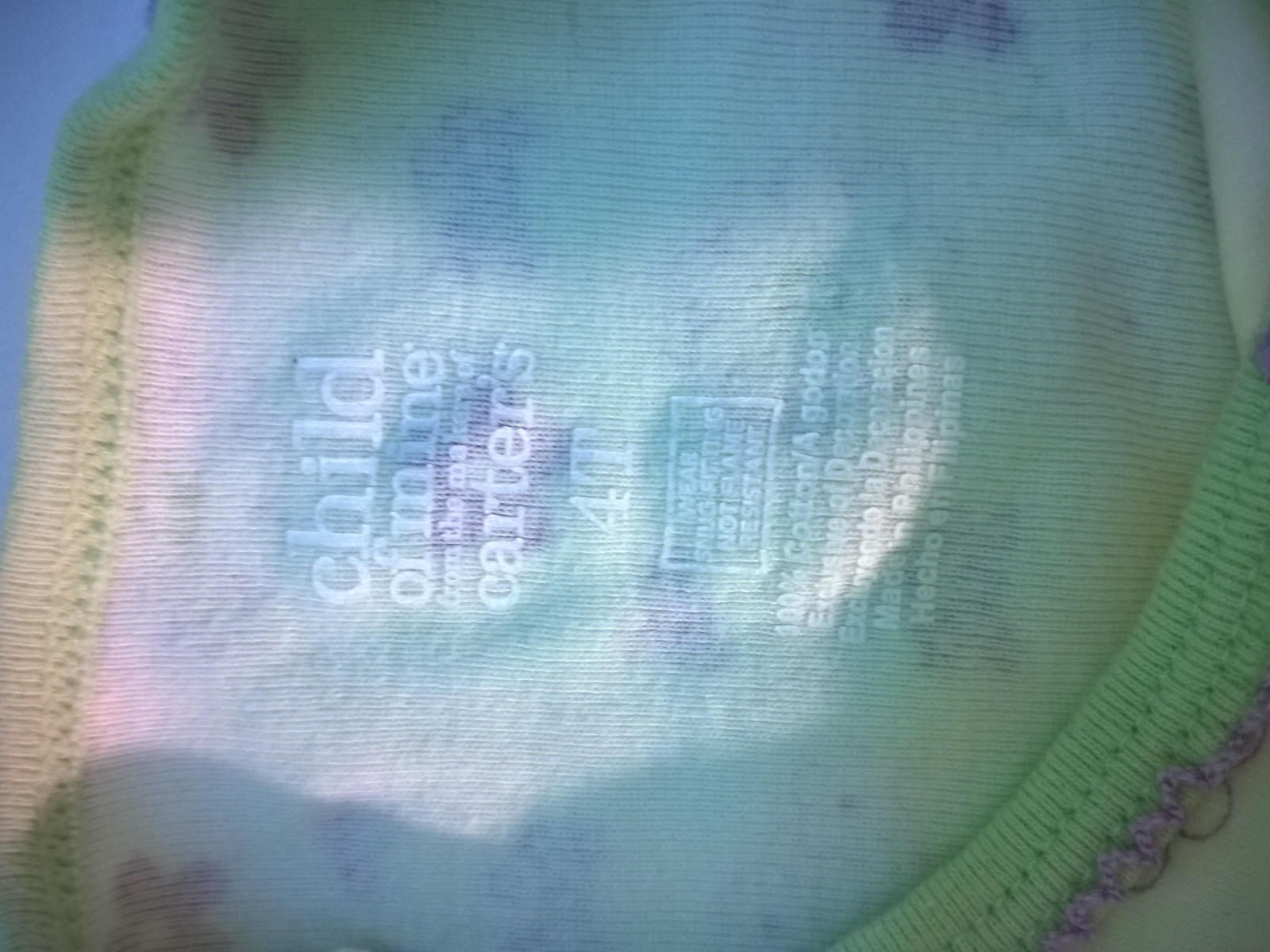The image is an extremely blurry, extreme close-up of a light-colored knit fabric, likely a young children's sweater or shirt. The knit texture is distinctly visible due to the close-up nature of the shot. The fabric appears to feature green and purple detailing around the edges, possibly including floral patterns with yellow centers. The garment's label, which is difficult to read against the pale yarn, indicates it is a "Child of Mine" product from the makers of Carter's, sized 4T, made from 100% cotton, and manufactured in the Philippines. The label also includes safety warnings about it being snug-fitting and not flame resistant, along with information in Spanish.